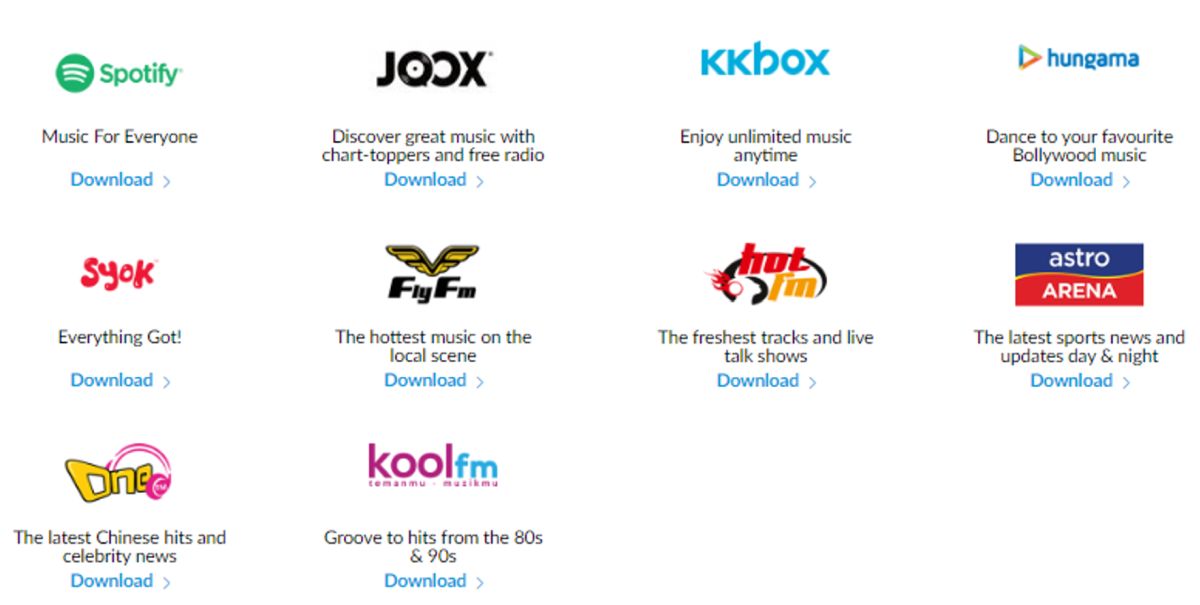The image features a white background divided into several sections, each showcasing a different brand logo and their respective taglines or descriptions. Starting from the top left, there is the Spotify logo with the tagline "Music for Everyone. Download." To its right is the JOOX logo, accompanied by the tagline "Discover great music with chart-toppers and free radio," with blue hyperlinks labeled "Download" under each.

To the right of JOOX, there's the KKBOX logo with the tagline "Enjoy unlimited music anytime." Continuing to the right, the Hungama logo appears with the tagline "Dance to your favorite Bollywood music." 

Below these, on the left, is the SYOK logo with a tagline suggesting comprehensive content. To its right is the flyFM logo, which boasts "The hottest music on the local scene." Next to it is the Hot FM logo, offering "The freshest tracks and live talk shows."

To the right of Hot FM is a blue and red box labeled Astro Arena, with the tagline "The latest sports news and updates day and night." Further down, next to this, is a section promoting "The latest Chinese hits and celebrity news."

Finally, at the bottom right, one last logo for Cool FM appears, with the tagline "Groove to hits from the '80s and '90s."